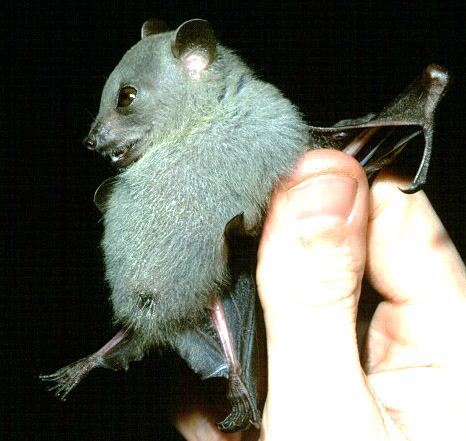This photograph captures a detailed close-up of a gray, furry bat being held by a person. The bat, with its small ears, short snout, and partially open mouth, stares off to the left. One of its feet extends forward, while the other foot appears tucked back toward the person's hand. The bat's wings are gripped, folded together between the thumb and index finger of the person's right hand, positioned at the bottom right of the image. The hand holding the bat is very bright, almost blown out, with visible details like the nail of the thumb. The bat's pink ear and its open eyes, which appear brown and black, add to the intricate details. The stark black background ensures that the bat is the focal point, standing out prominently in the photograph.